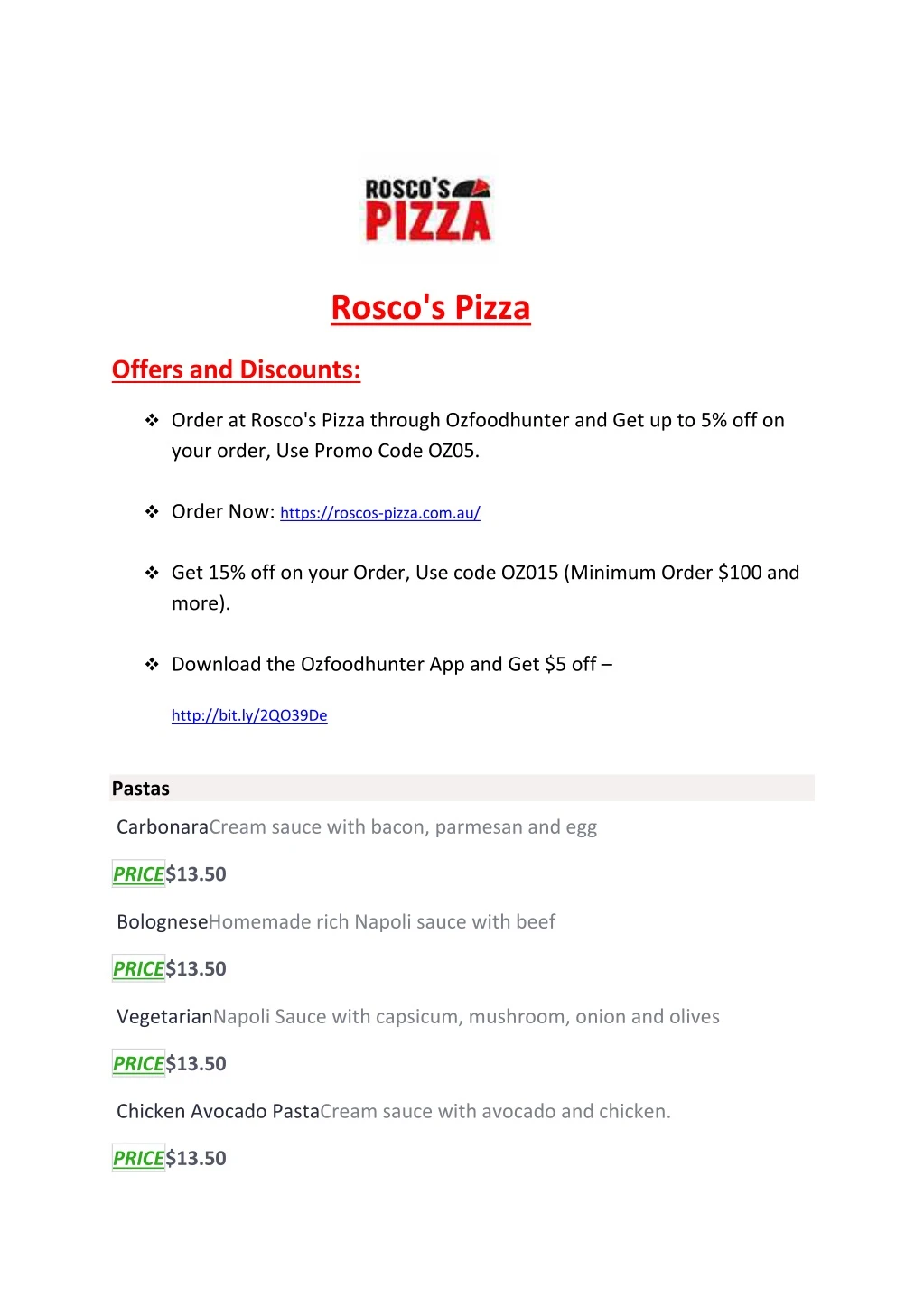**Website Screenshot Description:**

The screenshot showcases a website with a clean, white background. At the top center, the name "Roscoe's" is prominently displayed in black font. Directly below this, there is a black taco icon serving as a visual element.

Following the icon, the word "Pizza" is featured in large, bold red font. Subsequently, in underlined red font, the text reads "Roscoe's Pizza." Below this, another line in underlined red font states "Offers and Discounts:" introducing a bullet-point list.

The first bullet point, in black font, states: "Order at Roscoe's Pizza through Oz Food Hunter and get up to 5% off on your order, use promo code OZ05."

The second bullet point reads: "Order now: https://roscoes-pizza.com.au/"

The third bullet point, also in black font, details: "Get 15% off your order, use code OZ015 (minimum order $100 and more)."

The fourth and final bullet point in black font notes: "Download the Oz Hunter Food App and get $5 off - https://bit.ly/TQ039DE."

Below the bulleted list, there is a gray rectangle with the word "Pastas" in black font. Underneath, it describes a dish: "Carbonara cream sauce with bacon, parmesan, and egg."